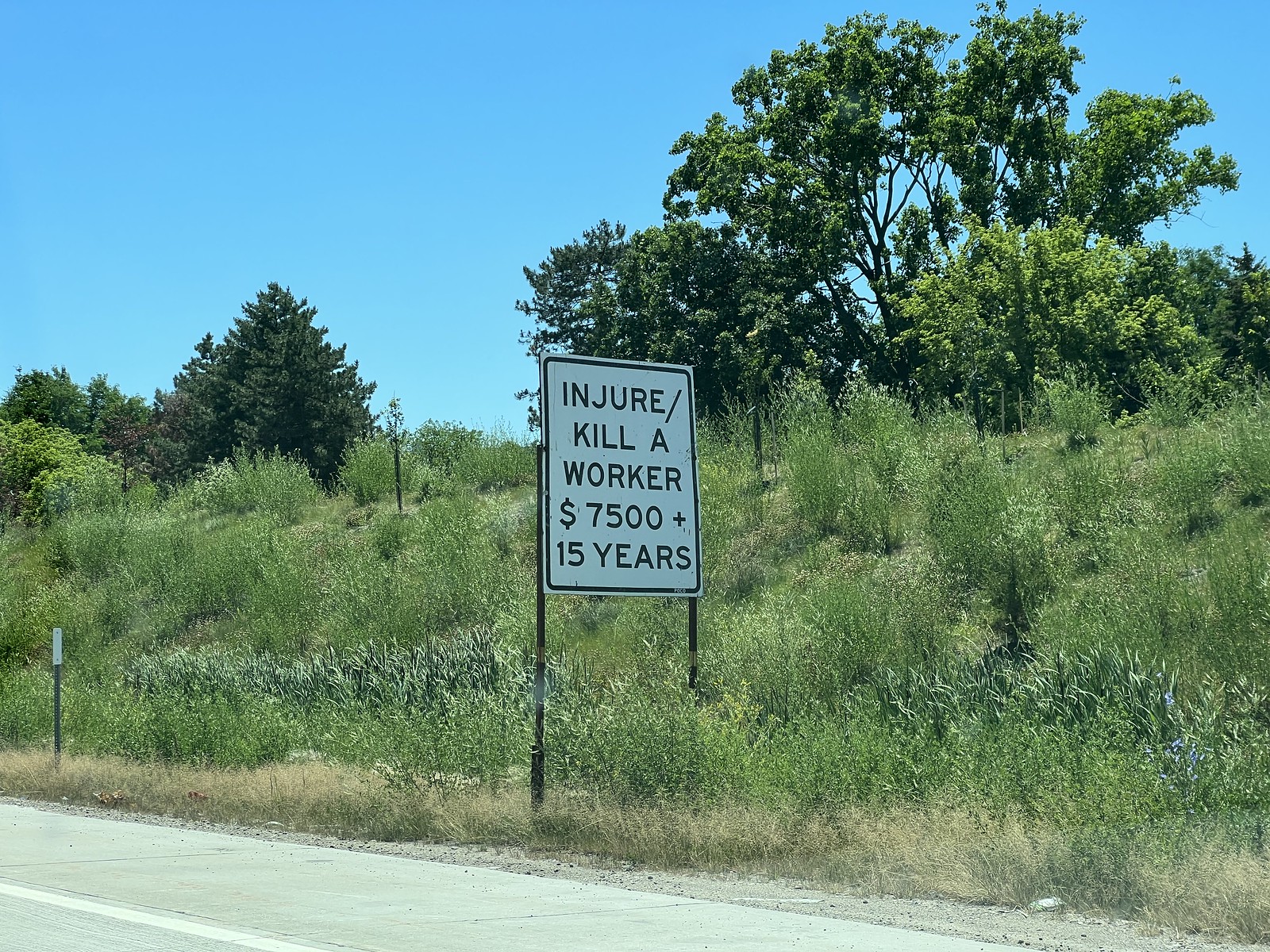This photograph captures a roadside scene dominated by a cautionary sign. The road itself enters the frame from the bottom left corner, featuring a gray surface marked with a crisp white lane line. Adjacent to the asphalt, a shoulder comprised of loose gravel transitions into a mix of short, dead grass. Progressing further into the background, a layer of taller, green grass and dense bushes can be seen. The landscape gently slopes upward to a small hill dotted with even larger bushes. Atop the crest of this hill stands a dense grove of trees, set against a sky of softly muted blue.

Prominently positioned in the center of the image is a stark white sign supported by two metal poles. The sign's shape is a rounded rectangle, and it bears a grave warning in black font: "Injure / Kill a Worker $7,500 plus 15 years." This message serves as a reminder of the severe consequences associated with reckless driving in work zones.